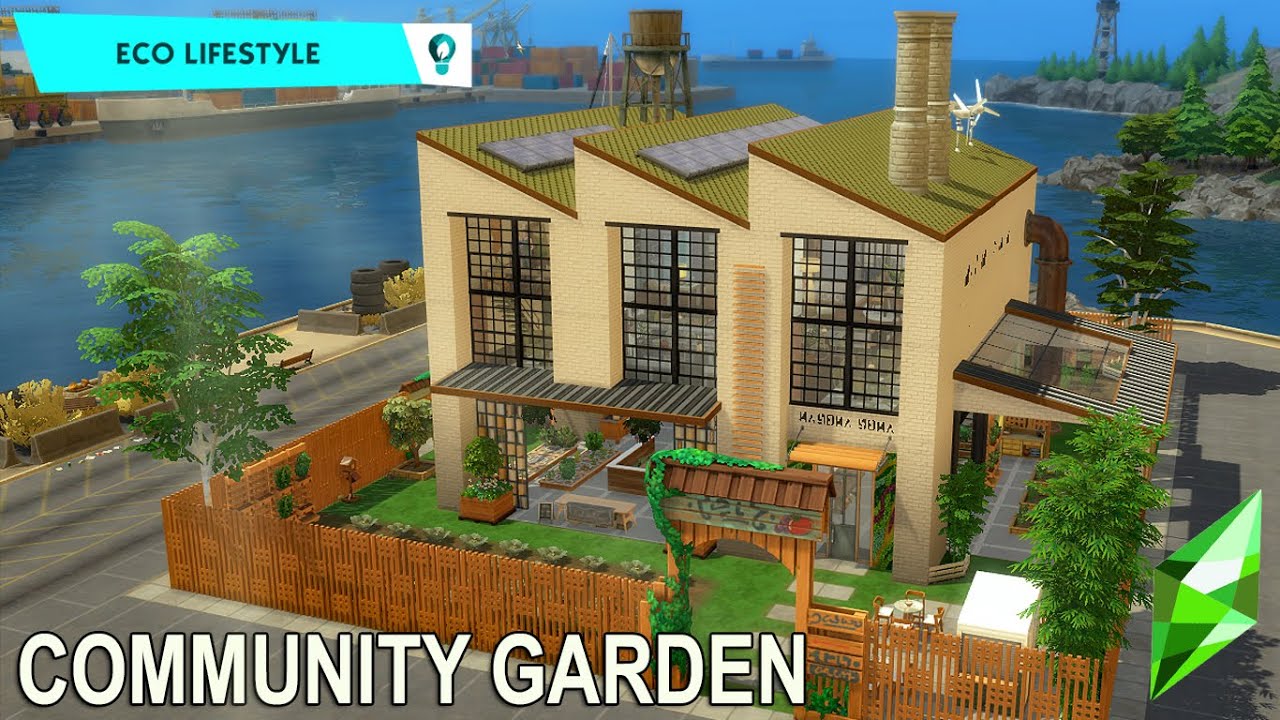This image is a computer-generated scene from the video game, The Sims, and showcases a community garden located at the edge of a body of water, likely near a harbor or dock. The garden is enclosed by a wooden picket fence and is fronted by concrete roads. The building within the garden appears to be a repurposed factory or an eco-efficient structure characterized by its sustainable features such as windmills, solar cells, and angled roofs. The beige building boasts an olive green jagged roof and has chimneys and other eco-architecture elements, including electric generators and a water tower. The bottom of the image features text in white letters reading "community garden," and the iconic green diamond from The Sims is visible in the lower right corner. In the distance, there are shipping containers being loaded onto ships, indicating the proximity to a shipping port. Additionally, the scene includes a few trees positioned at each corner of the square perimeter of the property, adding to its greenery. The top left of the image mentions "eco lifestyle" with the Nikon, highlighting the ecological theme of the setting.